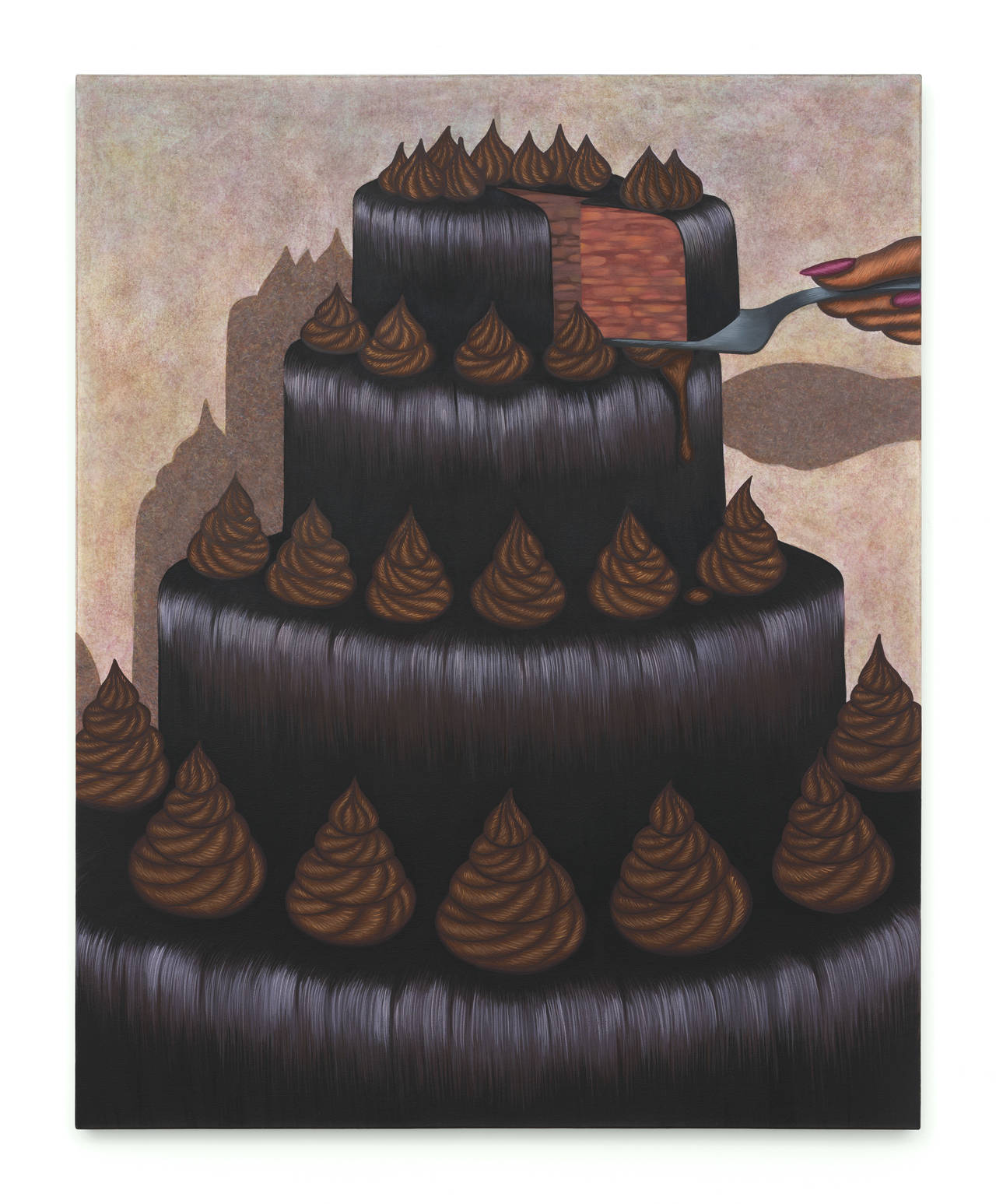This detailed artwork features a large, four-layered chocolate cake set against a mottled background of brown, tan, and gray hues. The cake, depicted in dark chocolate, showcases lighter chocolate dollops intricately placed around each layer, giving it a decorative appearance. A hand, dark in color, enters from the top right, using a silver utensil, possibly a spatula, to serve a slice from the top layer. The inside of the cake reveals a lighter, reddish-pink cellular texture, contrasting sharply with the glossy, almost hair-like exterior. The overall image evokes a surreal, almost unsettling vibe, further emphasized by the shadow casting off the cake.